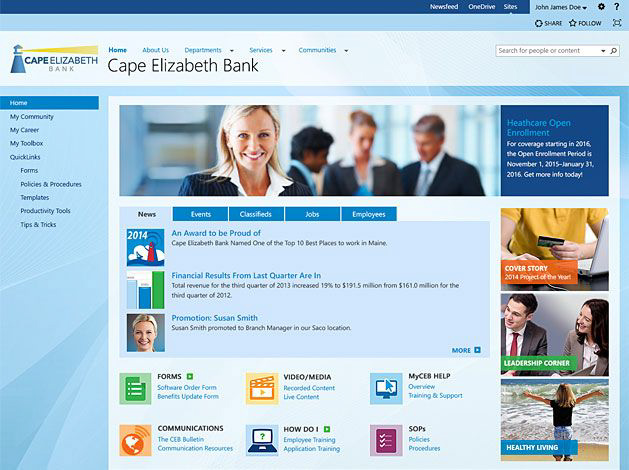The web page for Cape Elizabeth Bank is structured with a variety of sections and interactive elements, aimed at providing a comprehensive digital experience for its users. Positioned at the top of the page, the bank's name "Cape Elizabeth Bank" is prominent, flanked by different primary navigation tabs such as Home, About Us, Departments, Services, and Communities. Additionally, there are extra functionalities, including a search bar and buttons for sharing and following content. 

In the top-right corner, the name "John James Doe" appears beside icons for settings and help, indicating a personalized user area. The main navigation tabs highlighted in blue, specifically the Home tab, reinforces the user's current location on the site. Other tabs include My Community, My Career, My Toolbox, Quick Links, Forms, Policies and Procedures, Templates, Productivity Tools, and Tips and Tricks, providing a well-organized menu.

Notable updates and announcements are presented on the web page. One news item celebrates the accolade "Cape Elizabeth Bank named one of the top ten best places to work in Maine." Another update reveals significant financial results: the total revenue for the third quarter of 2013 increased by 19% to $191.5 million compared to $161 million for the same period in 2012. A third update announces the internal promotion of Susan Smith to branch manager at the SACO location.

The page also includes multiple sections for additional resources such as Forms, Videos and Media, My CEB Help, Communications, How Do I, and SOPs, offering users various informational materials. At the top of the page, a professional image features a woman in a business suit, with several people in the background engaged in conversation, presumably bank employees. Complementing the text, additional images related to finance enrich the visual appeal and context of the web page.